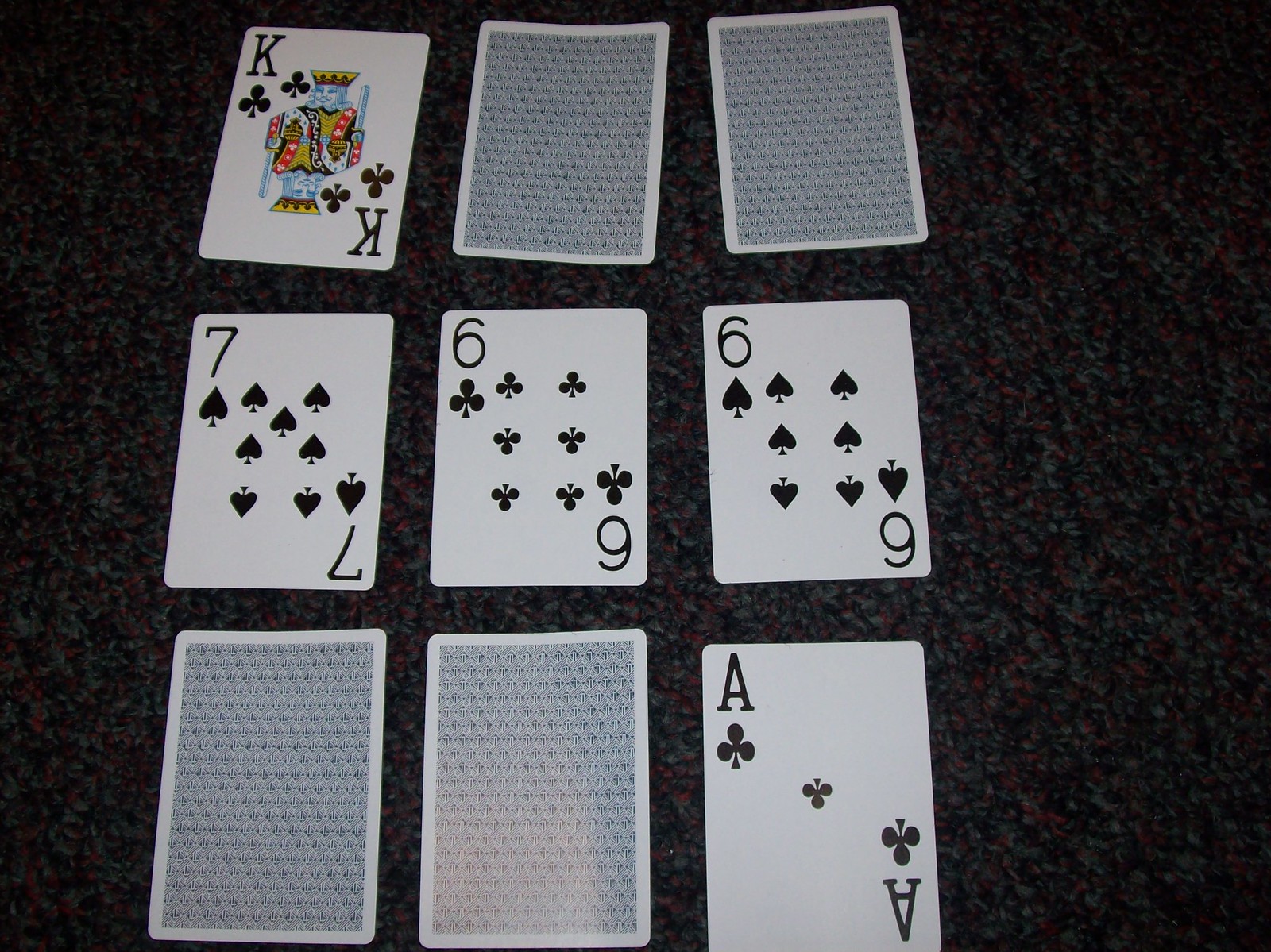In the image, a set of nine playing cards is arranged on a table in three rows of three. The cards have a navy blue back with a white trim design. Starting from the bottom row, the first and second cards are face down, while the third card is face up, revealing an Ace of Clubs. In the middle row, all three cards are face up; from left to right, they are a Seven of Spades, a Six of Clubs, and a Six of Spades. In the top row, the first card on the left is face up, showing a King of Clubs, while the remaining two cards on the right are face down. The intricate arrangement and the mix of face-up and face-down cards suggest that the individual is in the midst of a card game.